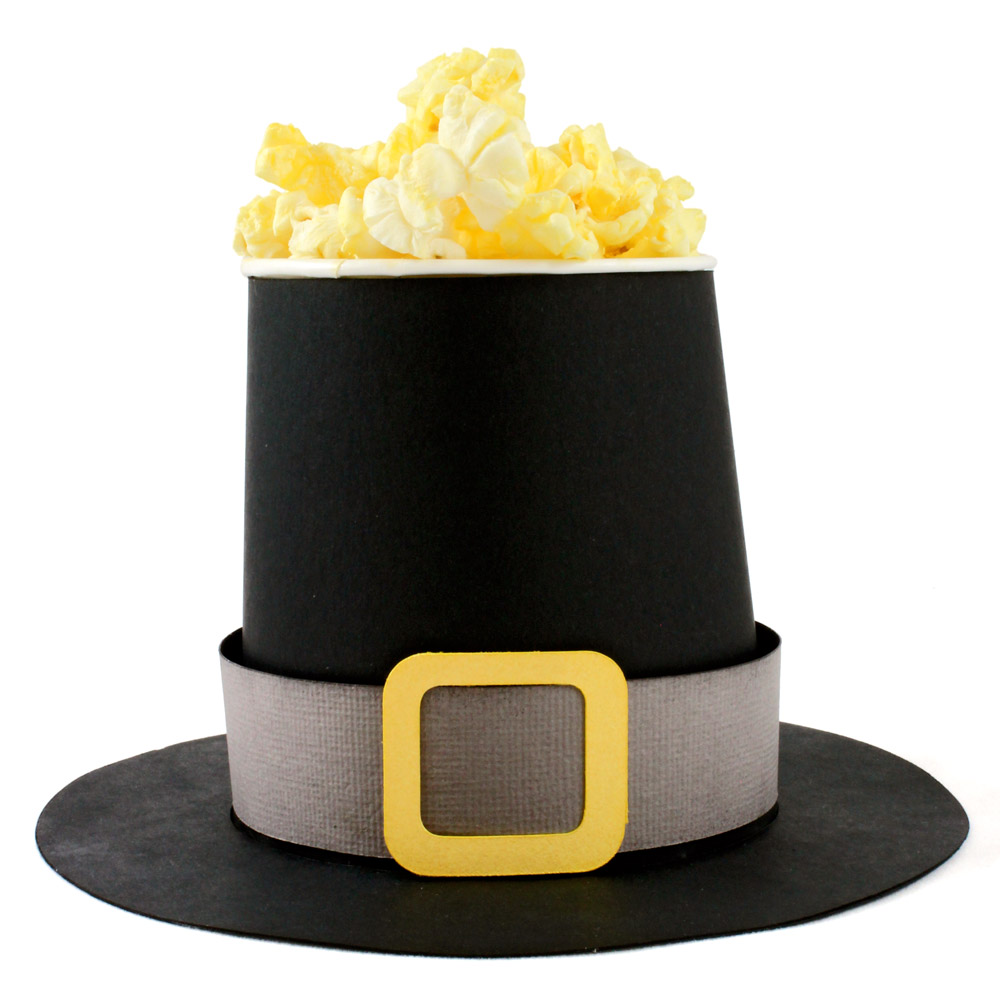The image features a detailed close-up of a black pilgrim's hat, complete with a traditional gray band encircling its base and a distinct gold square buckle with rounded corners on the front. The hat, crafted from felt, appears to repurpose as a whimsical popcorn bowl, with light, buttery-yellow popcorn spilling generously from its tapered top. Despite its charming appearance, the hat seems quite small, likely holding just enough popcorn for one person. The meticulously constructed pilgrim's hat, with its round brim and cylindrical top that tapers slightly inward, stands against a stark white background, emphasizing its festive, craft store aesthetic akin to a Thanksgiving decoration. Uniquely, the white rim of a popcorn bucket is subtly visible at the hat's opening, hinting at its playful conversion into a snack holder.